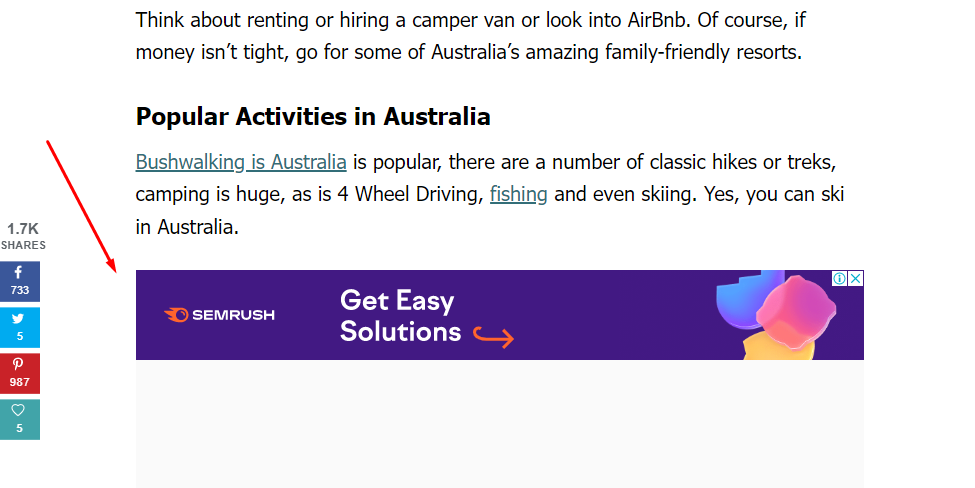Consider renting or hiring a camper van or exploring options on Airbnb for a flexible travel experience in Australia. For those with a more generous budget, Australia boasts some incredible family-friendly resorts. There are numerous popular activities to enjoy in Australia, with bushwalking being a favorite pastime. The country is home to many classic hikes and treks, making it a haven for outdoor enthusiasts. Camping is also very popular, as are four-wheel driving, fishing, and even skiing—yes, you can ski in Australia!

The image also includes various social media engagement metrics: 1.7k shares, with 733 on Facebook. There are also icons representing different platforms, including a blue square with a white bird (Twitter) indicating 1 share, a red square with a 'P' (Pinterest) showing 987 shares, and a teal square with a heart reflecting 3 shares. Additionally, a red arrow points to a purple banner with the text "SEMRUSH," along with a curved arrow suggesting "Get easy solutions." The far right of the banner features an emblem in blue, pink, and yellow, an information icon, and a small blue 'X' in the corner, likely representing a close button.